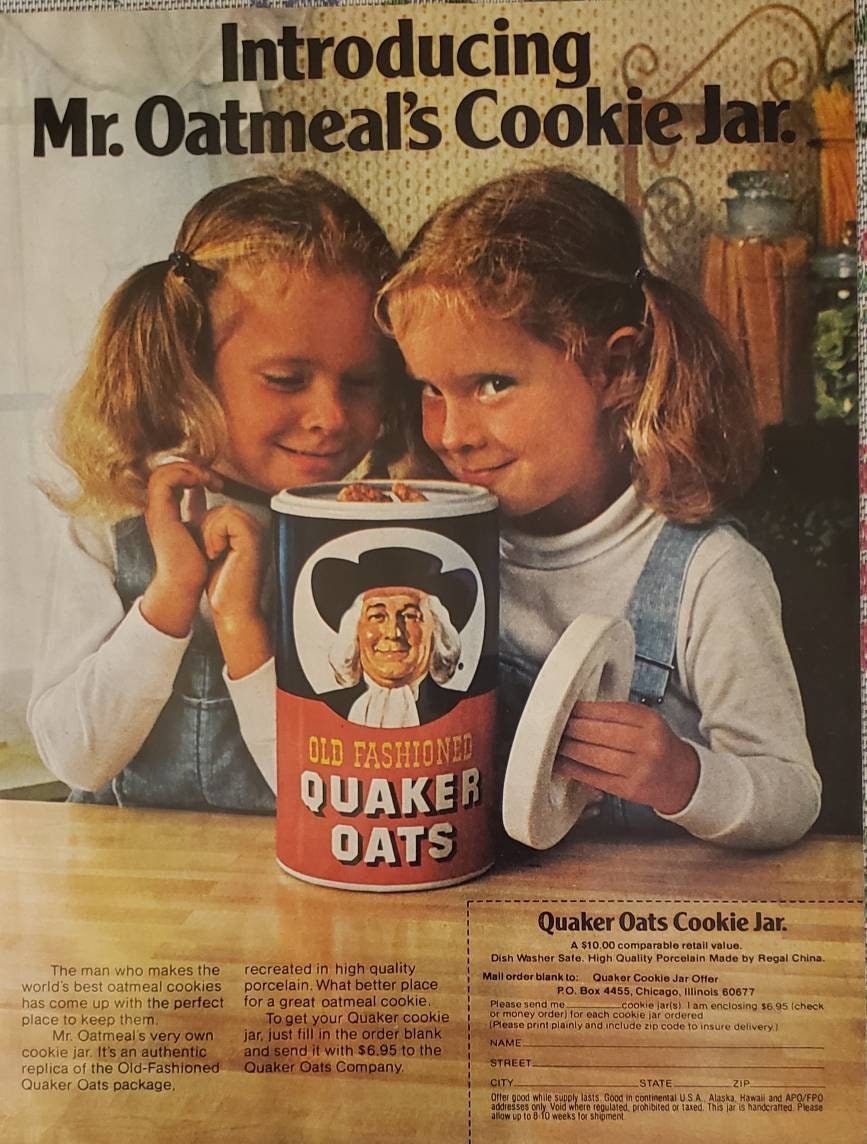This vintage advertisement from a magazine features two twin girls with blonde hair styled in pigtails, both garbed in white long-sleeved turtlenecks beneath blue jean overalls. The scene showcases an open Quaker Oats canister prominently placed on a wooden countertop, with the iconic Quaker man displayed on the front. One girl, brimming with excitement, gazes at the oatmeal canister, while the other, holding the canister lid in her left hand, wears a mischievous expression.

Above them, bold black text reads, "Introducing Mr. Oatmeal's Cookie Jar," hinting at the true content within the canister – cookies, not oatmeal, which explains their joy. The Quaker Oats package, in blue and red with a white lid, is described as having an authentic replica jar available for purchase. The bottom of the ad details the offer: "The man who makes the world's best oatmeal cookies has come up with the perfect place to keep them. Mr. Oatmeal's very own cookie jar is an authentic replica of the Old Fashioned Quaker Oats package, recreated in high-quality porcelain. Order yours for $6.95."

The ad features additional promotional details on the right, including the price of $10 for the cookie jar, marked as dishwasher safe and crafted by Regal China. The surroundings include a metal shelf on the right with jars of red, green, and orange items, a white curtain to the left, and brown and tan wallpaper on the right.